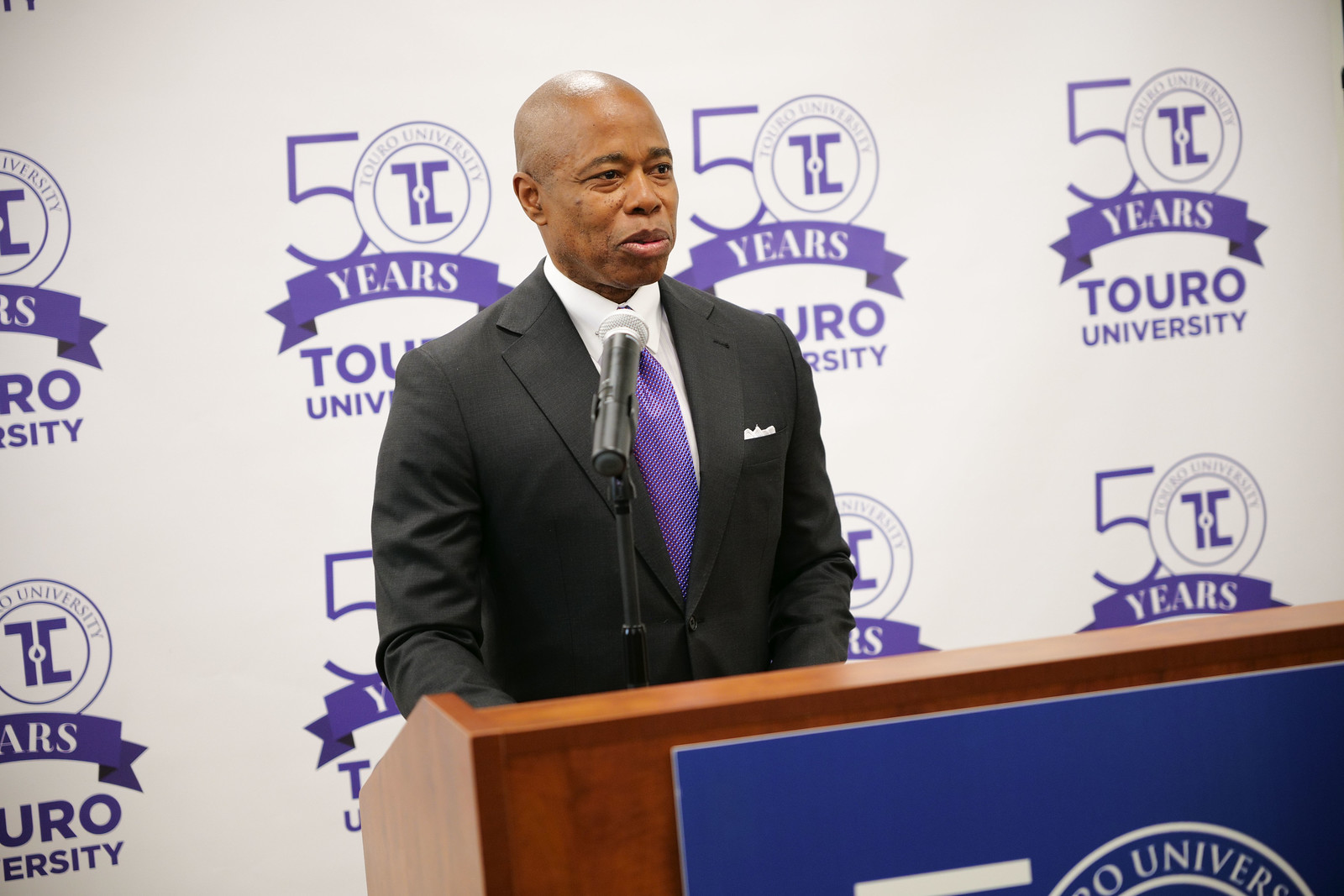This image features Mayor Adams of New York City, an African-American man with a bald head and brown skin, delivering an official speech at Touro University. He stands behind a light brown wood podium emblazoned with the university's logo, speaking into a microphone. Mayor Adams is elegantly dressed in a black suit paired with a checkered black and white tie, a white shirt, and a white pocket square. The backdrop behind him prominently displays the logo "50 Years Touro University" in shades of blue, brown, blackish gray, and white, with the word "years" stylized as a ribbon, repeating multiple times across the white background. This detailed setting suggests that the event is likely a significant celebration, possibly a graduation or an anniversary marking Touro University's 50th year.